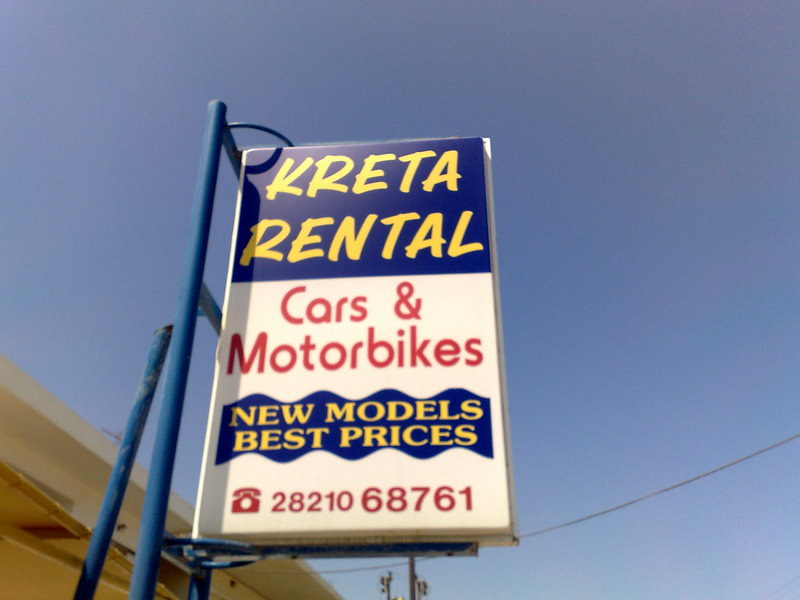This image captures an outdoor commercial sign for "Creta Rental" from a lower angle, accentuating the sign against a brilliant blue sky. The sign is mounted on a blue post and is vertically rectangular in shape. The upper portion of the sign features a dark blue background with yellow text that reads "Creta Rental, K-R-E-T-A Rental." Below this, a white section with red text advertises "Cars and Motorbikes." Further down, the sign showcases a wavy dark blue area with yellow writing that reads "New Models, Best Prices." At the bottom of the sign, a small red telephone icon is accompanied by the number 28210-68761. Behind the sign, an electrical or phone wire stretches across the scene. In the lower left corner, the edge of the light-colored building is visible, enhancing the commercial setting of the image.